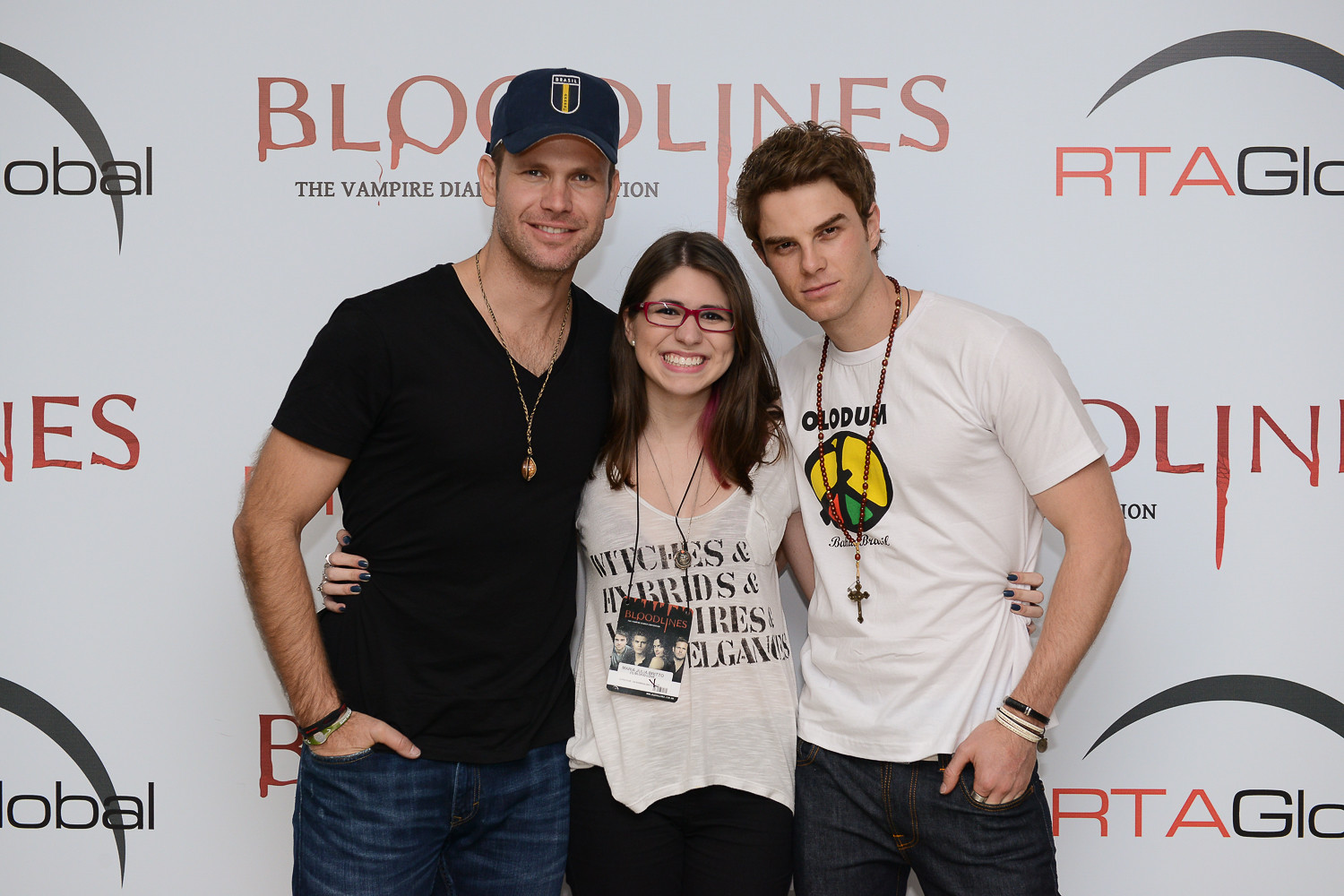In this photo, three Caucasian individuals are posing in front of a white backdrop with repeating logos and text, including "Bloodlines: The Vampire Diaries" and various sponsors. The man on the left sports a navy blue ball cap, a black V-neck t-shirt, a long wooden necklace, blue jeans, and two bracelets. His right hand rests in his pocket, and he has dark eyes. The woman in the center, with shoulder-length brown hair and red-framed glasses, is beaming. She wears a loose-fitting v-neck t-shirt featuring the words "witches and hybrids," partially covered by a lanyard displaying a Vampire Diaries tag, as well as dark pants. Her arms are around the waists of the men on either side of her. The young man on the right has short brown hair and wears a white t-shirt with a central design likely incorporating a peace sign. He accessorizes with a rosary-like necklace and bracelets on his left hand, completing his look with dark blue jeans.